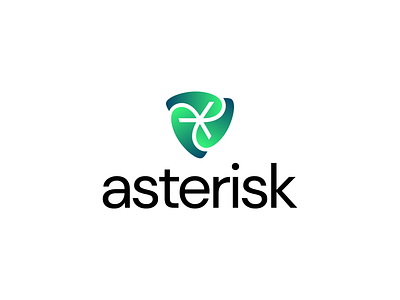The image features a completely white background with a centrally positioned logo that has a gradient of green tones, transitioning from a bright, light green at the center to a darker, deeper green at the edges. The logo resembles an abstract, curvy triangular shape, reminiscent of a guitar pick or fig, with three interlocking teardrop-like or yin-yang shapes forming a cohesive, circular pattern. At the center of this logo, there's a white asterisk. Directly beneath the logo, the word "asterisk" is written in lowercase black font, clearly legible even at a distance.